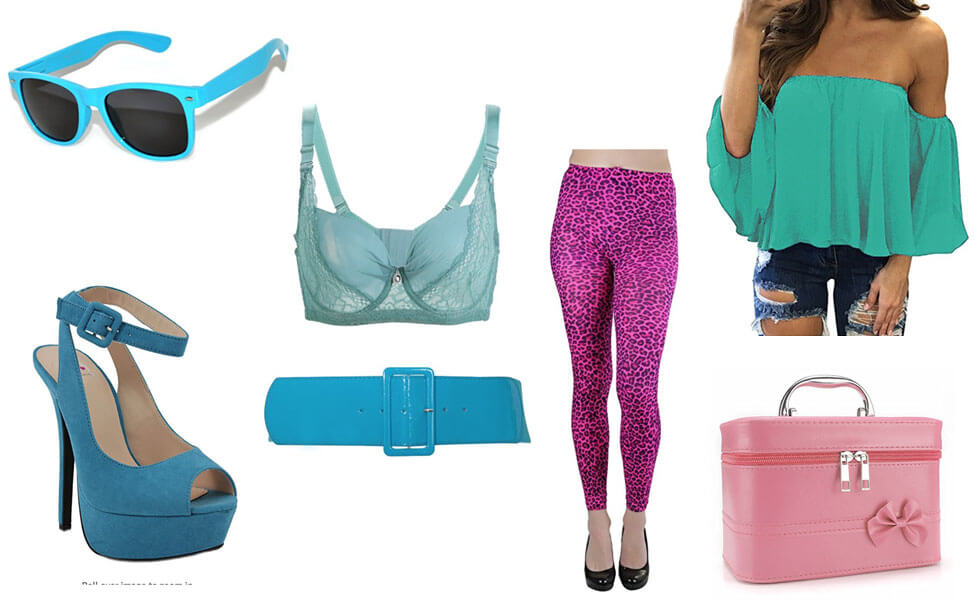This image showcases a vibrant collection of women's accessories set against a white background. Starting from the upper left corner, the striking aqua-colored sunglasses with dark lenses immediately catch your eye. Below them is a stylish light blue bra, paired with a darker blue vinyl belt. Moving further down, a pair of high-heeled platform shoes stands out with their deep blue color and black spiked heels. To the right, a bright greenish-blue blouse with ruffled sleeves adds a touch of elegance. Adjacent to it, purple leggings with a black leopard-like pattern bring a pop of boldness. Finally, a compact pink handbag with a silver handle and intricate zipper details complements the ensemble, adding functional fashion. Altogether, these items present a colorful and trendy outfit, indicative of a careful and creative selection of accessories.